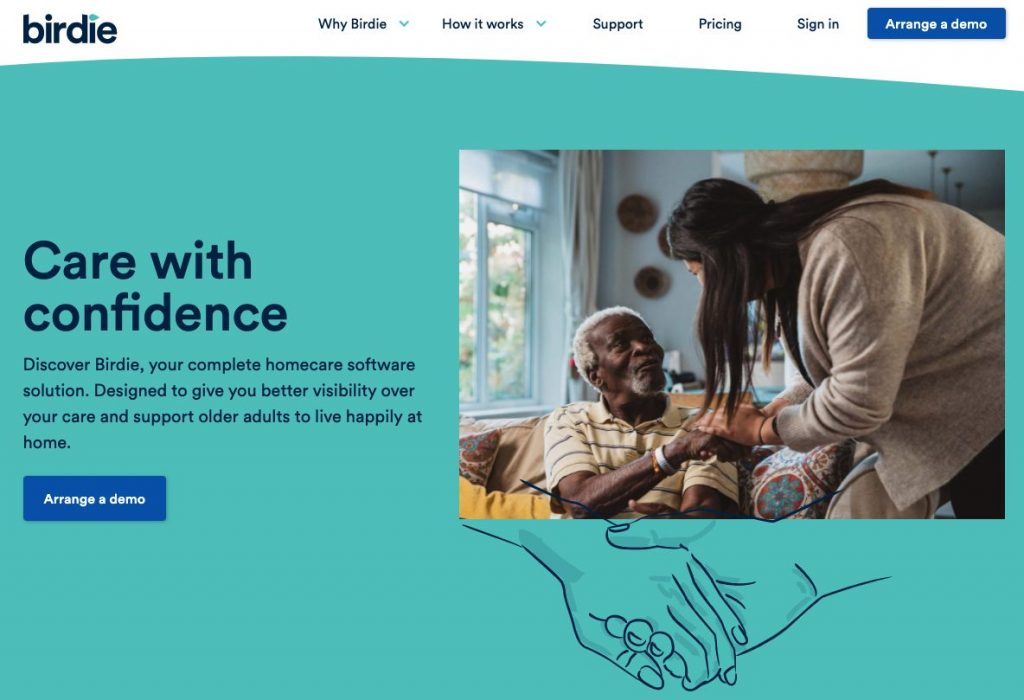The image depicts the homepage of a website named "Birdeye," spelled B-I-R-D-I-E. The logo features the unique detail of a small bird perched atop the letter "i," integrated into the dot above the "i." Central to the image is a heartwarming photograph of an elderly person seated, holding hands with a younger caregiver in a gesture of support and assistance. The scene beautifully conveys compassion and care.

To the left, text prominently reads "Care with Confidence," followed by a detailed description: "Discover Birdeye, your complete home care software solution designed to give you better visibility over your care and support older adults to live happily at home." Directly beneath this text is a noticeable blue button with white text that reads "Arrange a Demo," inviting users to click and schedule a demonstration of the software.

Across the top of the website are several submenus offering additional information and navigation options. These include:
1. "Why Birdeye" with a dropdown arrow indicating more options.
2. "How it Works," which also suggests further selections.
3. A "Support" link.
4. "Pricing" information.
5. A "Sign In" button.
6. Another "Arrange a Demo" button located in the top right corner for easy access.

This comprehensive and user-friendly layout ensures that visitors can effortlessly explore Birdeye's offerings and find the support they need.